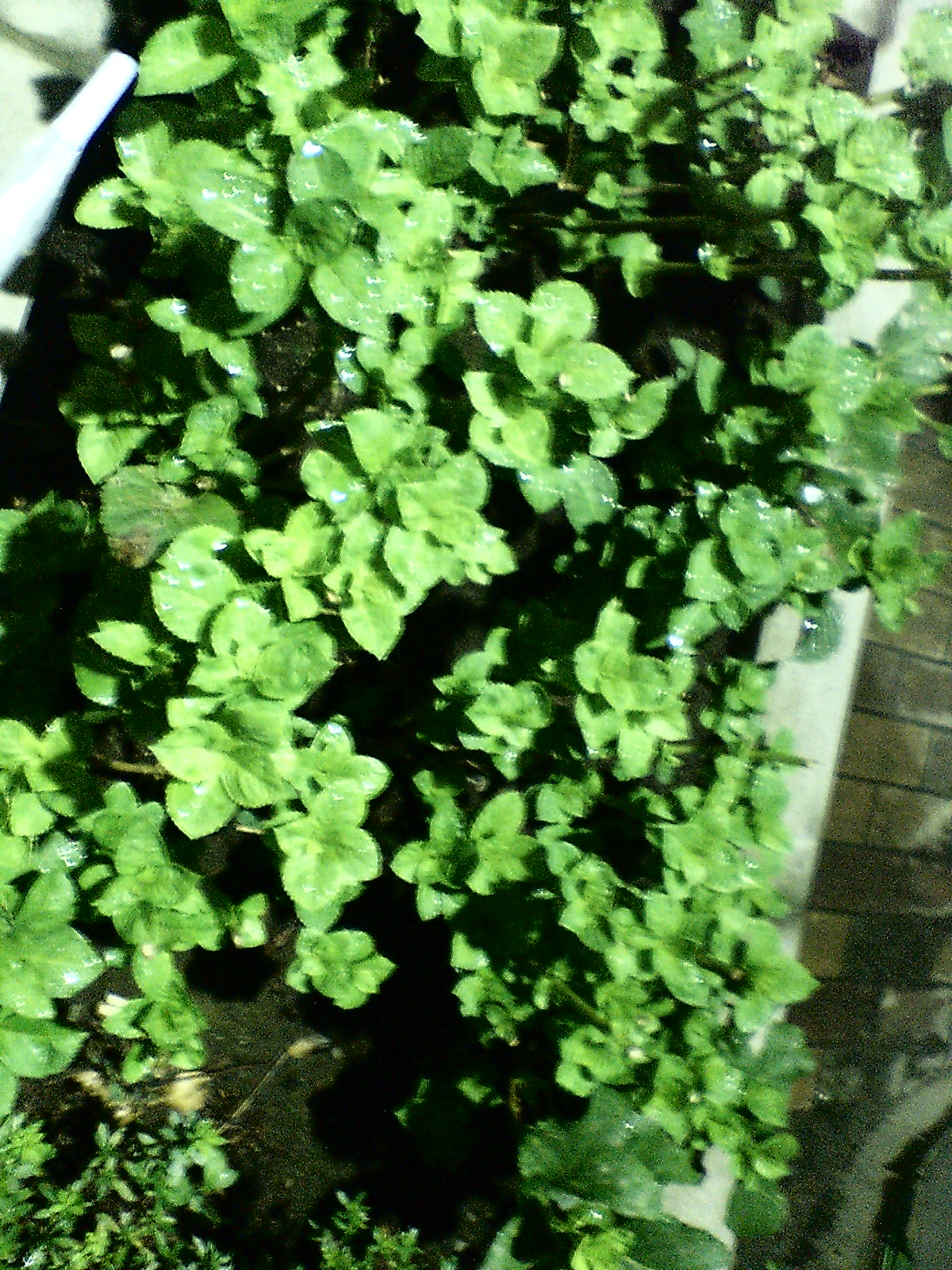This grainy and blurry photograph appears to be an old, low-quality close-up taken outdoors. It predominantly features a mass of green foliage, possibly potted plants or a bush, with leaves of a lime green hue. Some of the leaves are speckled with what seems to be dew droplets. The plants are set against the side of a building, as indicated by a white downspout emerging from the structure and a background of clay or tan-colored bricks to the right. The vantage point suggests the photo was taken from above, looking down on the plants. There's also a hint of soil and some smaller flowers at the base of the foliage. Despite the blurry nature of the photo, the vivid green of the plants is the most striking aspect.